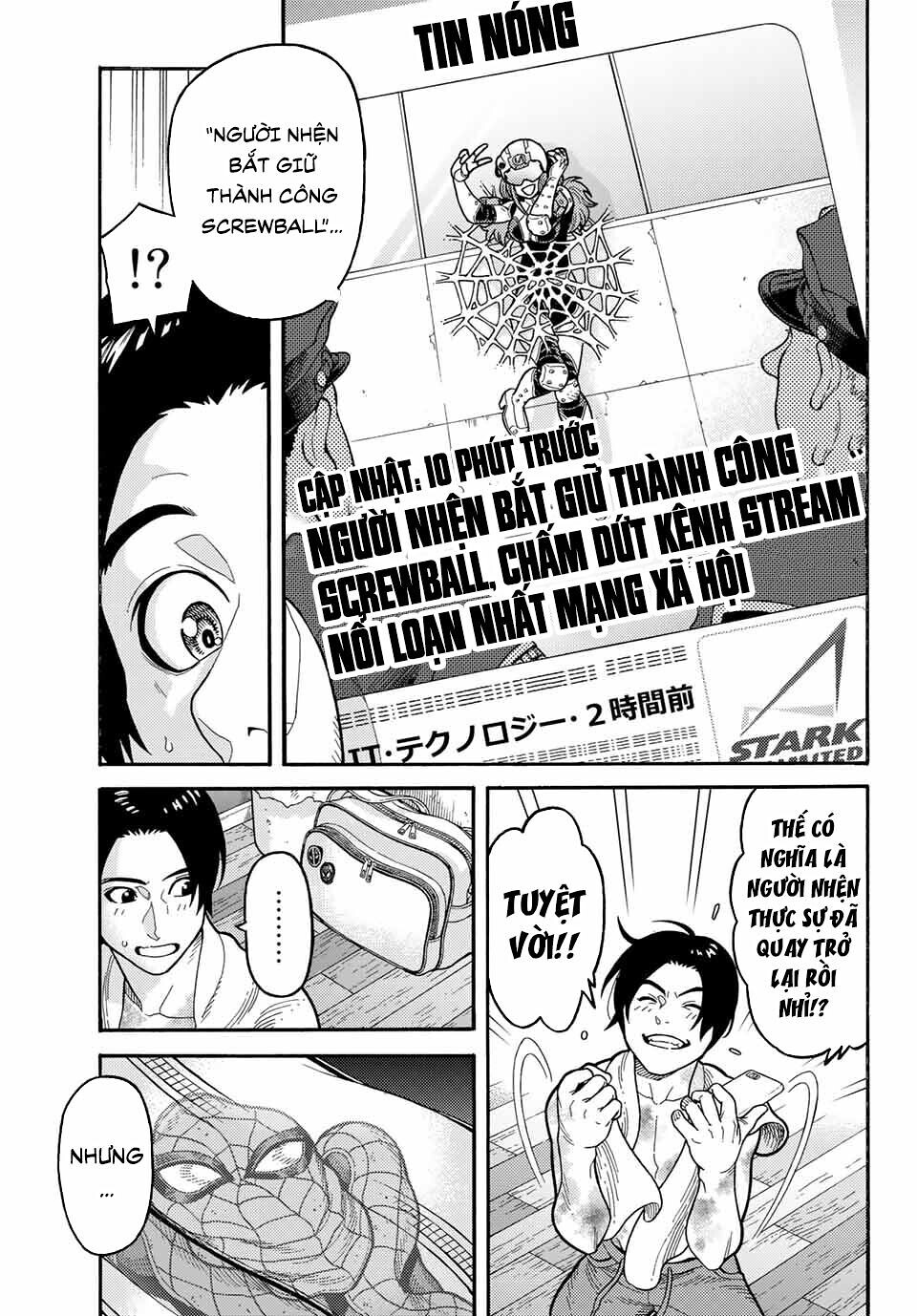This black and white comic strip, resembling a Japanese manga, is composed of six panels arranged in a grid. The very top left panel, a narrow sliver, features a close-up of a startled character's eye with black hair and an unreadable thought bubble in a foreign language. To its right, the second panel shows a person, seemingly immobilized by Spider-Man's web, trapped against a wall. Two police officers stand nearby, observing the scene, with the word "screwball" visible amidst foreign text. Below, on the left, the third panel depicts a man glancing over his shoulder at a suitcase. Beneath it, the fourth panel shows a Spider-Man-like figure from a top-down perspective, looking upwards. The final panel on the bottom right captures the same man as earlier, now kneeling on a wooden floor and pulling his shirt off with a broad smile on his face. All the dialogue and text in the comic strip are in an unreadable language, adding a layer of mystery to the scenes.